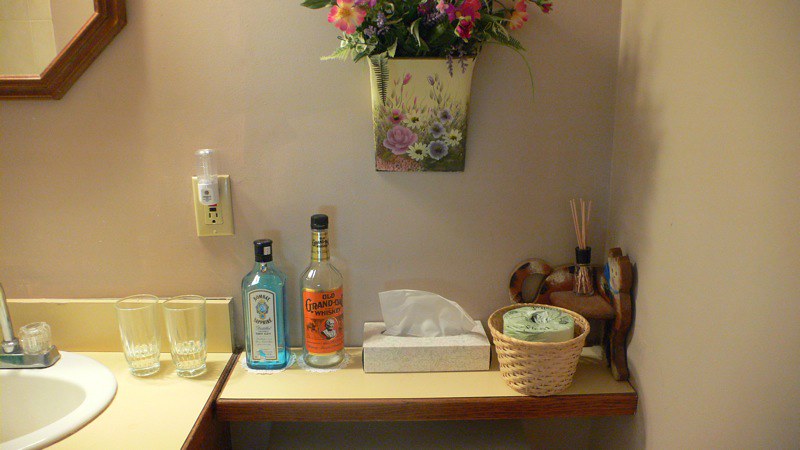The image depicts a cozy bathroom scene showcasing a partial view of a bathroom vanity and adjacent shelving, adorned with various items. The vanity, made from pale yellow laminate with a wooden border, features the left third of an oval white sink equipped with a faucet that includes a crystal-like knob and a tall chrome spout. Two clear water glasses, partially filled to roughly one-third, rest on the vanity surface, which stands against a pinkish-white wall.

Above the vanity is a grounded wall socket housing a nightlight. The room boasts an octagonal mirror with a detailed wooden border, of which only the bottom quarter is visible in the top right corner of the image. 

To the right of the vanity, a similarly designed shelf holds a bottle of Bombay Sapphire Gin and an Old Grand-Dad Whiskey bottle, both of which appear to be empty. Next to these bottles is a box of Kleenex with an accessible tissue, an unopened roll of green tissue paper in a wicker basket, and a white diffuser jar with bamboo sticks resting on a cat-shaped wooden shelf. This quirky shelf wraps around a corner, creatively utilizing both the back and side walls for a unique decorative touch.

Hanging above the shelf is a square planter-like object, painted with an array of pastel flowers, and filled with artificial blooms, including begonias, hydrangeas, and green foliage, providing a touch of nature and color to the bathroom setting.